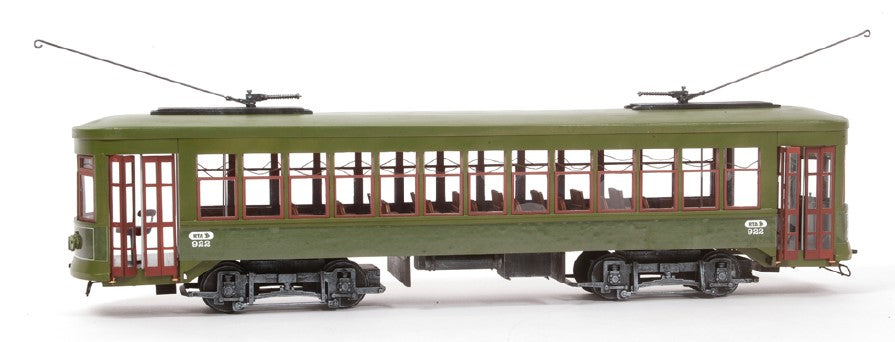This detailed image showcases a meticulously crafted model of a streetcar set against a clean, white background. The streetcar, painted in a soothing army green, is highlighted with dark, stained wood trim around its numerous windows and doors. At both ends of the car, there are functional glass-paneled, double-folding doors painted in a light rusty red, designed to open for passenger entry and exit. The model features realistic detailing, including interior benches for passengers and standing handles. The conductor's area, identifiable by a single seat facing the front, is clearly visible. The roof of the streetcar is equipped with two cables extending upwards, designed to connect to a power source, mimicking the operation of a full-size trolley. The streetcar rests on eight detailed black wheels, suggesting it would typically run on tracks. This model captures the essence of a historical streetcar with intricate craftsmanship.